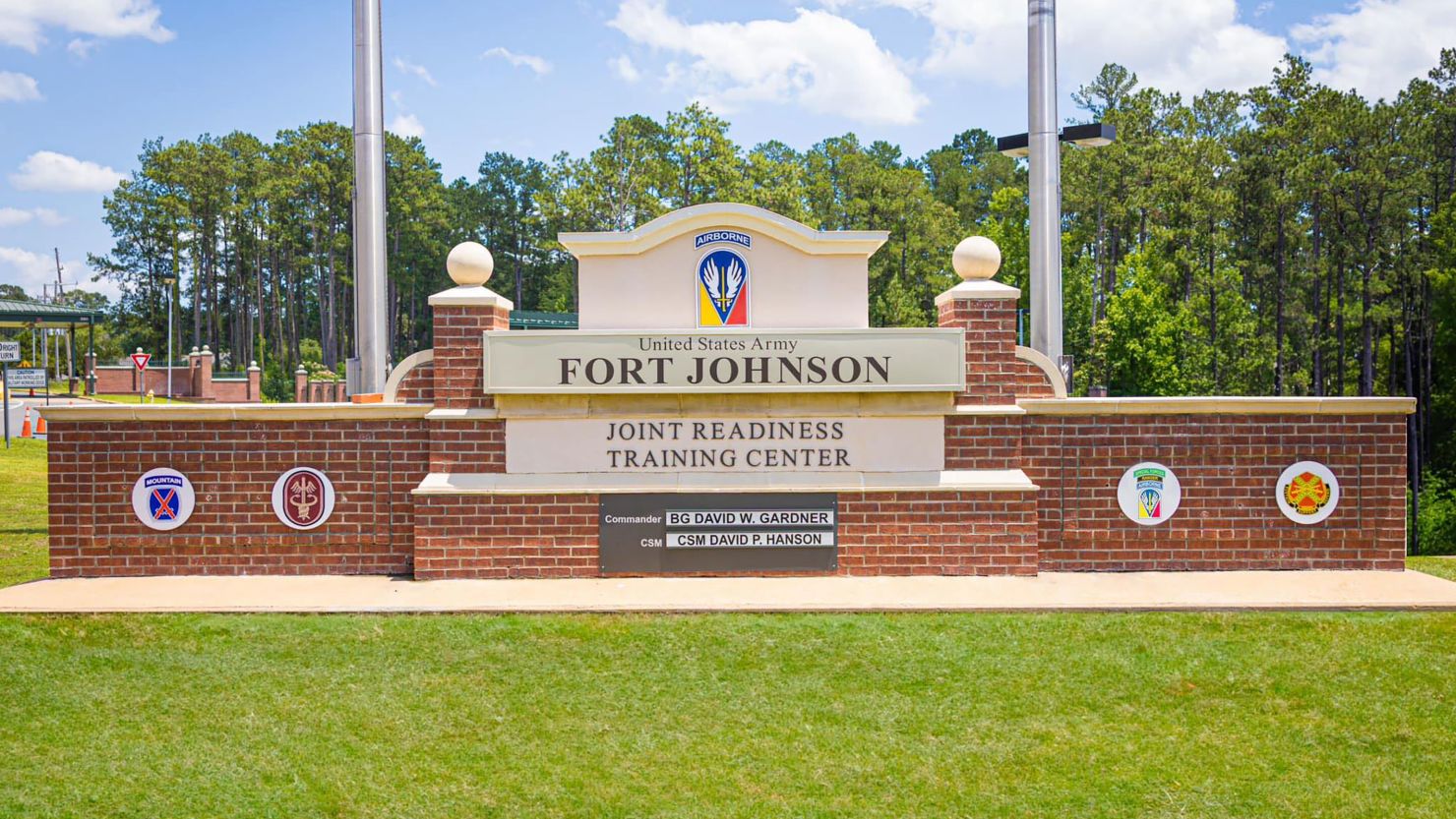This is an image of the United States Army Fort Johnson Joint Readiness Training Center's prominent brick structure sign, situated outside the facility to signify its presence. The sign features two tall, silver, round metal poles, one equipped with lighting, flanking a central brick plinth adorned with a cream-colored cement cap. In the middle of the structure, there's an arched roof with the text "United States Army" in smaller font and "Fort Johnson" in larger, black lettering, prominently displayed beneath. Below this, on a cement slab, it reads "Joint Readiness Training Center," and further down, in darker gray, are the names "BG David W. Gardner" as the commander and "CSM David P. Hansen" as the CSM.

To the left of the waist-high brick wall, capped with cement, are two insignia: one featuring a blue circle with crossing swords on a pinkish-red background and another dark red and yellow circle with what appears to be an eagle and a sword. Additional circular insignia in teal, orange, and white can be seen, contributing to the display's significance. The foreground is adorned with a neatly maintained lawn, and the background features trees and a glimpse of other brick structures, likely part of the training center. The sky above is blue with clouds, adding to the overall dignified and authoritative appearance of the sign, which serves more as a memorial or grand entrance marker rather than a mere directional sign.